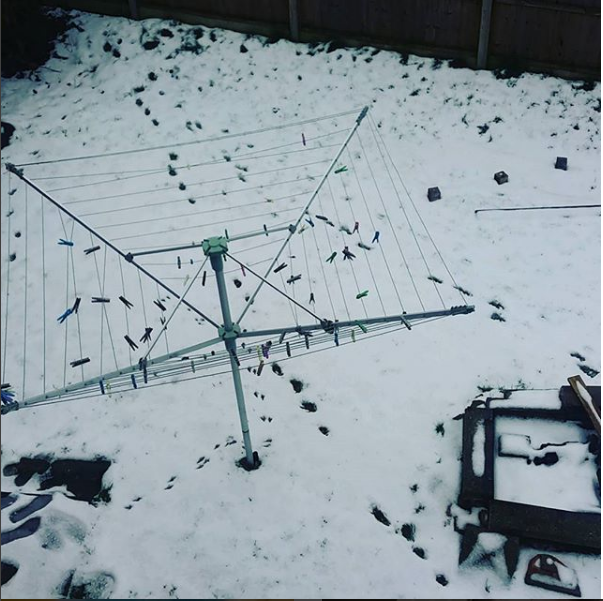This black-and-white image captures a serene, snow-covered yard viewed from a second-story window. The entire yard is blanketed in a pristine layer of snow. Along the fence line, which is slightly visible, a cluster of bushes is situated in the upper right corner. Dominating the center of the yard is an old-fashioned, square-shaped clothesline, standing tall with multiple tiers of wire lines, each adorned with a scattering of clothespins. Footprints crisscross the snowy expanse: tiny prints likely made by birds or squirrels meander around the base of the clothesline, while more sizable human footprints carve distinct paths through the snow. A set of slightly larger tracks—possibly from a dog—traverse the yard, adding to the story of this winter scene. In the foreground, a box-like structure is also enshrouded in snow, its function obscured by the wintry blanket. This bird’s-eye view offers a tranquil snapshot of a snow-laden backyard, filled with signs of life despite the chill.